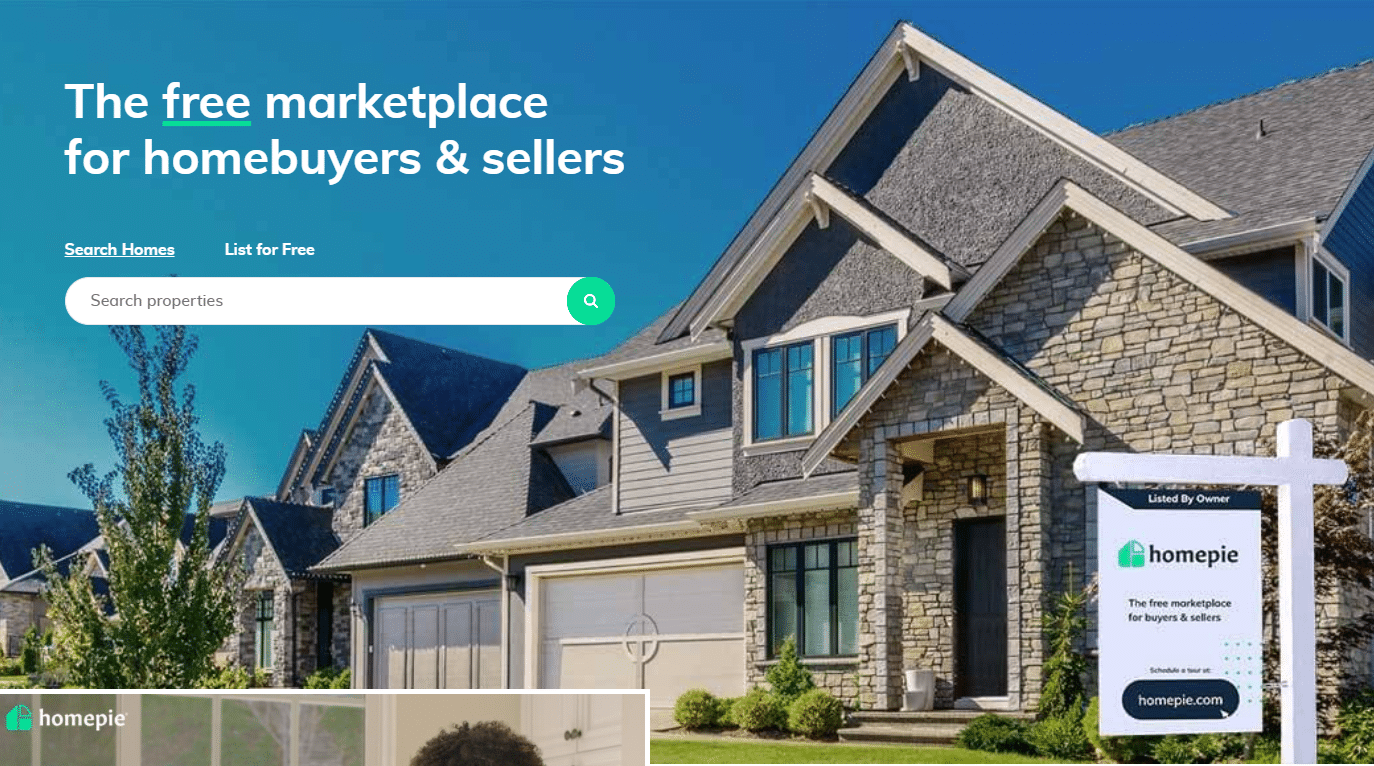Caption: 

The landing page of the HomePi website presents a visually striking background image of an expansive, multi-million dollar brick home, featuring multiple angled roofs, two prominent garage doors at the front, and a stone facade. The soft, natural lighting illuminates the scene from the upper left, enhancing the grandeur of the residence.

In the upper left corner, overlay text in white reads "The free marketplace for home buyers and sellers." The word "free" is underlined with a clean, horizontal green line for emphasis. Beneath this, a slogan encourages users to "Search homes, list for free," accompanied by an inviting, horizontal search bar.

On the lower right side of the image, a signboard stands out, displaying the HomePi name and the tagline, reinforcing the website's purpose. The HomePi logo is also visible in the lower left corner, rendered in white lettering next to a sleek, modern icon. 

This inviting and intuitive landing page sets the stage for visitors to explore HomePi's offerings seamlessly.